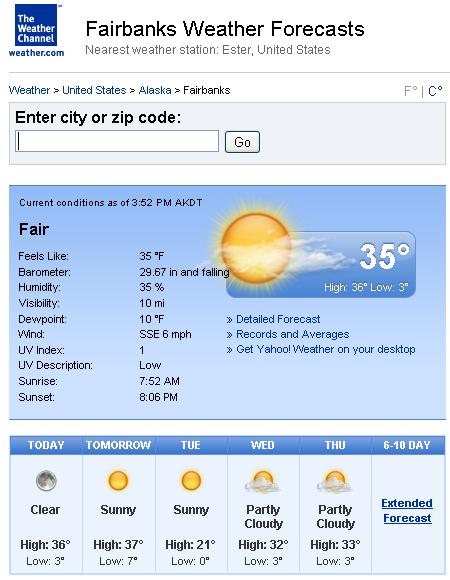Certainly! Here is a cleaned-up and detailed caption:

---

This image shows a detailed weather forecast on the Weather Channel's website for Fairbanks, Alaska. The background is predominantly white, with the Weather Channel's signature blue icon positioned in the upper-left corner, next to the text "weather.com" written in blue.

To the right of the icon, in larger font, it reads "Fairbanks Weather Forecast," with the smaller text beneath, "Nearest weather station: Ester, United States." Below this heading, a thin gray line spans the width of the page.

On the far left, small blue text indicates the navigation path: "Weather > United States > Alaska > Fairbanks." On the far right, there is an option to toggle between Fahrenheit and Celsius, with Fahrenheit selected.

Beneath this section, there is a gray banner where users can change locations by entering a city name or zip code in a white input box accompanied by a "Go" button.

The main content area features a large blue box displaying the current weather conditions. At 3:52 PM AKDT, the conditions are noted as "Fair." Several weather metrics are listed below, including "Feels Like," "Barometer," "Humidity," "Visibility," and "UV Index." On the right side of this box, there is an image depicting the sun with a few clouds, suggesting partly sunny skies. The temperature is 35°F, with a high of 36°F and a low of 3°F.

Under this main forecast box, there are links for "Detailed Forecast," "Records and Averages," and an option to "Get Yahoo Weather on Your Desktop."

A light blue rectangular box follows underneath, featuring a darker blue banner at the top. This section outlines the extended daily weather forecast, including "Today," "Tomorrow," "Tuesday," and "6 to 10 Days," with descriptors of expected conditions such as sunny skies along with high and low temperatures for each day.

---

This detailed caption ensures a clear and comprehensive understanding of the webpage's layout and content.